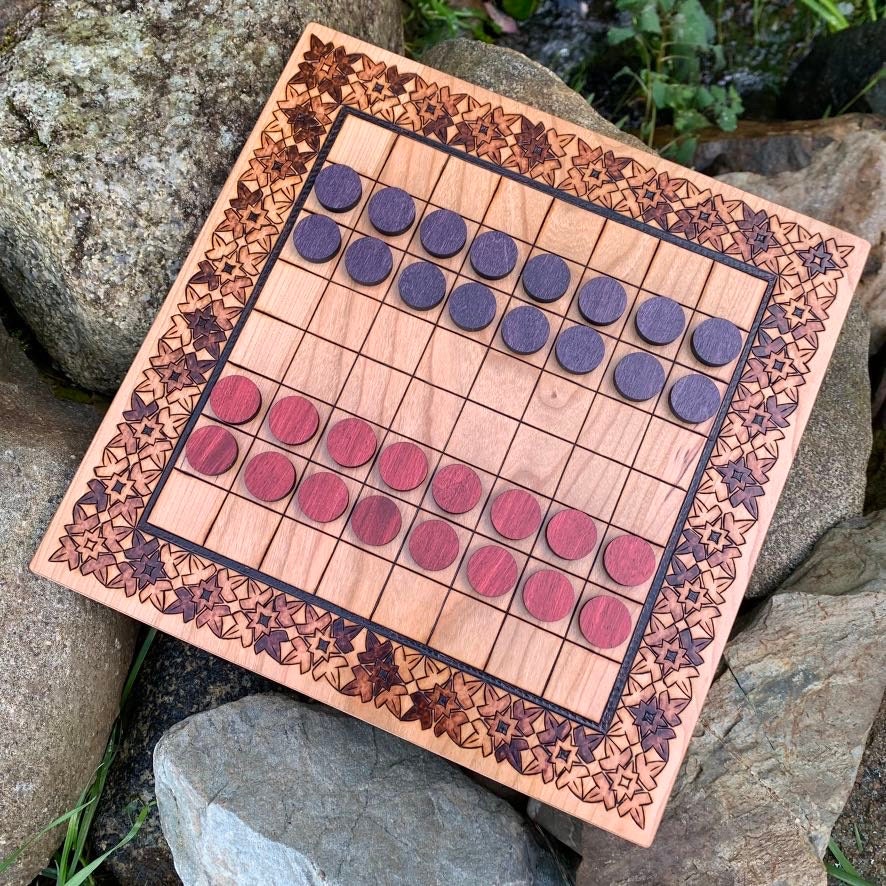This photograph captures a wooden checkerboard with a polished, lacquered finish, featuring a floral and decorative design around its edges. The board is positioned at a slant, tilted approximately 30 degrees to the right, and is set atop a bed of football-sized grey rocks with brown speckles and some green foliage visible in the background. The checkerboard itself has red and black checkers strategically placed; there are 16 red checkers lined up in rows towards the bottom and 16 black checkers towards the top, each set beginning from the second row, leaving a single empty row behind them and two empty rows in between the opposing colors. The floral designs around the perimeter appear intricately laser-cut into the wood, adding an elegant touch to the overall scene.